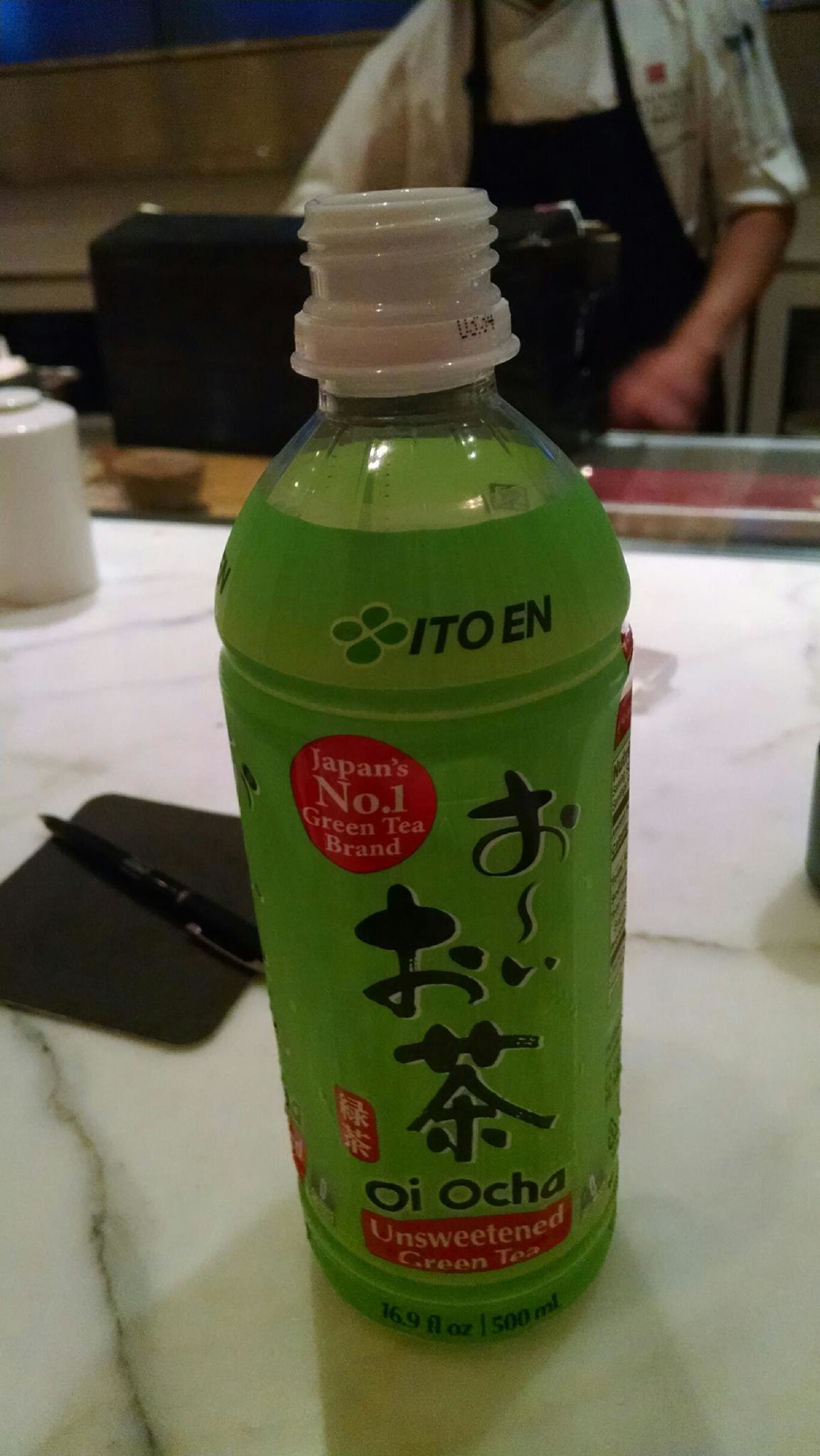In a cozy kitchen with blue walls and light brown cabinets, a person is focused on cooking, dressed in a brown apron over a white shirt with rolled-up sleeves. A radio sits nearby, playing in the background. Dominating the foreground is a large, white table with subtle black streaks. On the table, there is a black notepad, a black pen, and salt and pepper shakers. Also noticeable is a green bottle with a white cap, labeled "Ito En." The bottle features a red circle with the number one, along with the text "Oi Ocha" and black Chinese characters, as well as another small red detail.